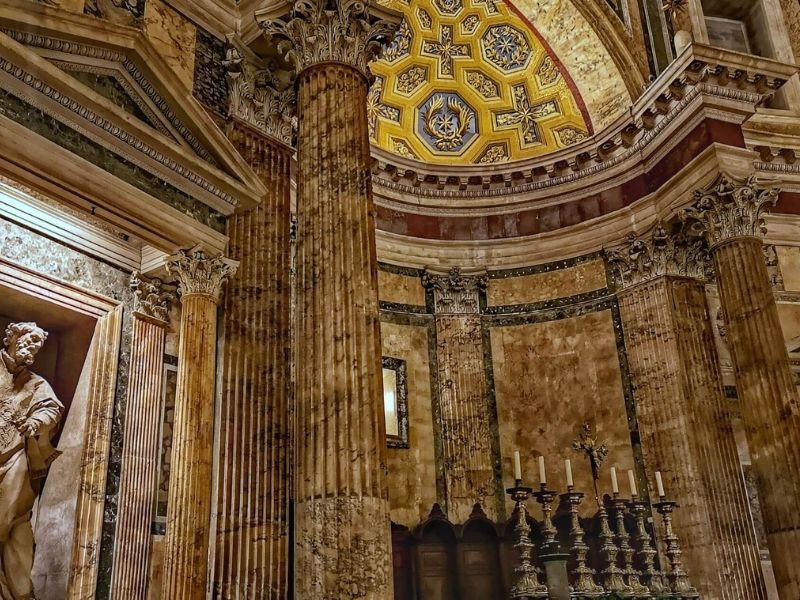The image captures the interior of a grand cathedral with towering cathedral ceilings adorned with intricate designs. The primary hues inside the cathedral are various shades of brown and beige, while the ceiling features vibrant yellow, gold, and blue details. The ceiling is richly decorated with engravings, including crosses, stars, angel-like wings, and octagonal or sextagonal shapes. The dark brown pillars ascend impressively from floor to ceiling, contributing to the grandeur of the space.

In the lower left corner of the picture, there is a statue of a religious figure situated within an alcove that has a doorway-like frame. Above this alcove, a sloped roof-like structure in brown with light green accents can be seen. At the bottom foreground, there are six white candles arranged in holders placed symmetrically around a central crucifix. This scene is set against a backdrop of brown marble walls with dark brown ornate facades underneath the gold ceiling details. The entire structure exudes a sense of historic elegance and solemnity.